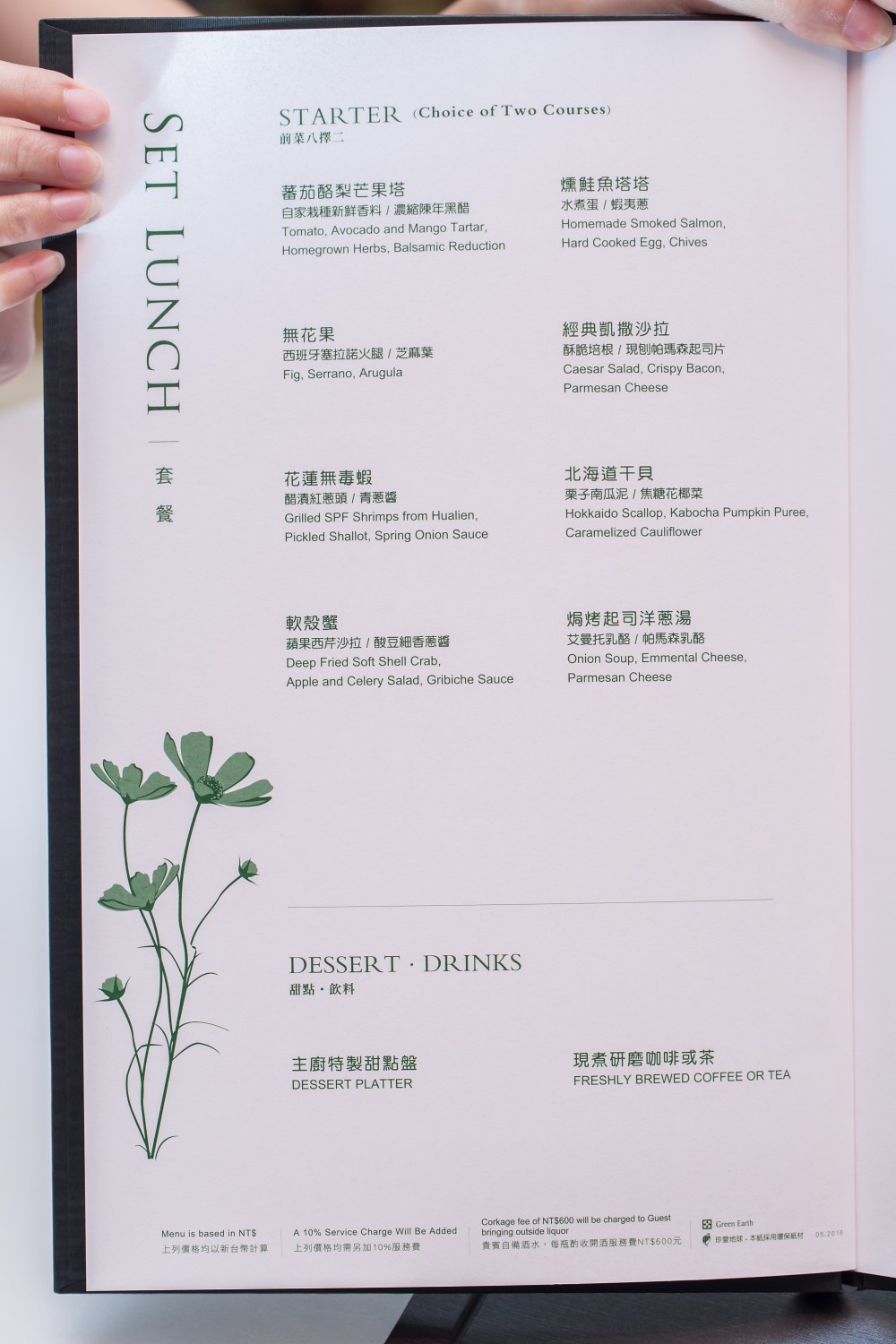The image features a color photograph of a restaurant menu being held and displayed toward the camera. A woman with elegantly manicured, slender fingers is holding the menu, her four neatly positioned fingers visible at the top left corner, while her thumb is obscured behind the menu. Her left hand, partially visible in the top right corner of the frame, pushes the menu open to ensure it stays unfolded.

The menu itself is printed on white paper and is adorned with a simple yet charming illustration of wildflowers, depicted in green ink. The illustration features three blooms and a couple of buds supported by slender stems with narrow leaves. Though the name of the flower eludes the observer, it is identified as a yellow flower commonly found in their garden.

The menu's categories are organized under "Set Lunch" followed by Chinese characters. The title at the top of the menu lists "Starter," "Choice of Two Courses," though the finer details are too small to discern clearly. The text, which alternates between Chinese characters and English translations, is printed in a dark green font. Despite the small print size, the observer manages to identify a section dedicated to "Dessert and Drinks" at the bottom of the menu. This section mentions a "Dessert Platter" with accompanying Chinese characters, and to its right, more Chinese characters precede the words "Freshly Brewed Coffee or Tea." 

The overall presentation is simple yet elegant, capturing the artistic illustration and neatly formatted menu items, although the finer print remains largely unreadable due to its size.